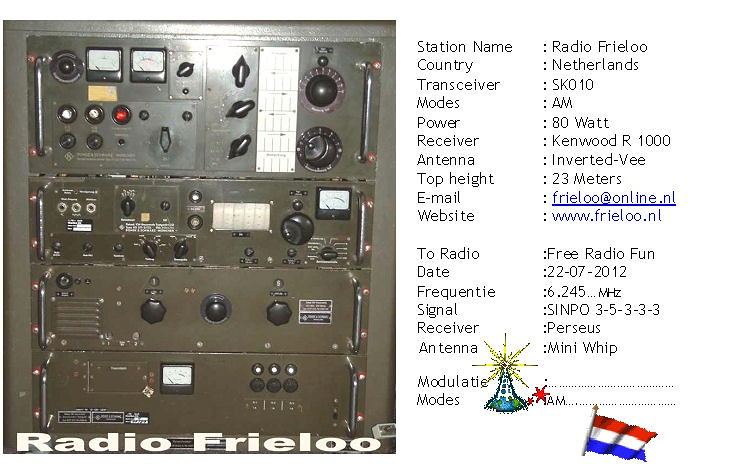The image predominantly features a photograph covering the left half of the page, depicting old radio equipment with a dark brownish-green hue and silver metal handles running vertically along its sides. The equipment is adorned with numerous dials, knobs, and gauges, and carries the white text "Radio Freeloo" at the bottom. The right side of the page contains a description box detailing the system. The station name is Radio Freeloo, located in the Netherlands, utilizing an SK010 transceiver and Kenwood R1000 receiver, with a power output of 80 watts and an inverted V antenna at a top height of 23 meters. Detailed specifications include the frequency 6.245 MHz, signal strength SINPO35333, and the date 22-07-2012. Contact information is provided: email freeloo@online.nl and website www.freeloo.nl. Additionally, the bottom section displays the French flag and a radio tower emoji. The overall appearance of the radio device suggests it may be a reprint of an older image, with intricate black and white controls giving it a vintage look.